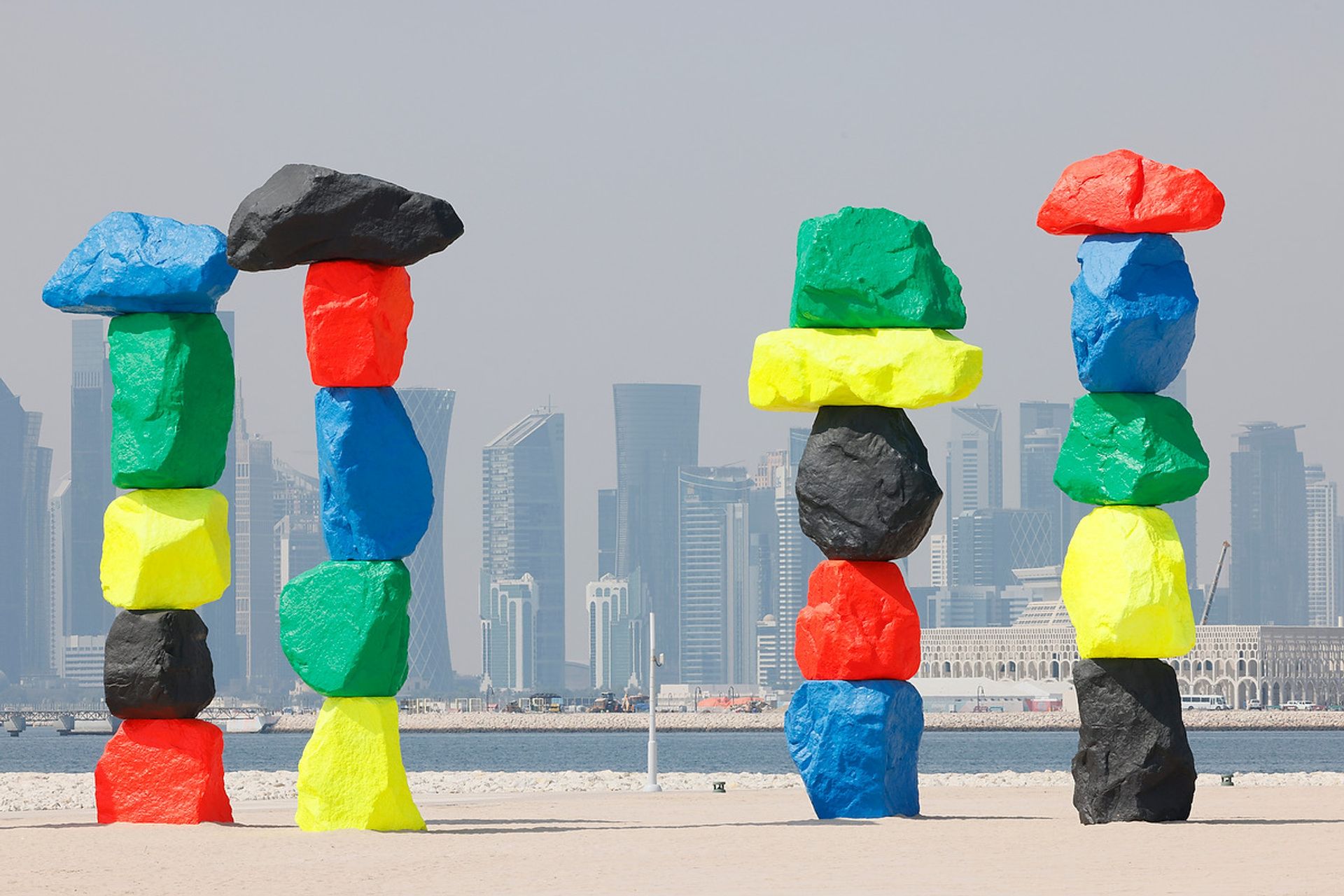This image appears to be a creative combination of drawing and photography, showcasing four towering stacks of vividly painted rocks in the foreground. Each stack consists of five large rocks in different colors: blue, green, yellow, red, and black. From left to right, the stacks are ordered as follows:

1. Blue on top, followed by green, yellow, red, and black.
2. Black on top, followed by red, blue, green, and yellow.
3. Green on top, followed by yellow, black, red, and blue.
4. Red on top, followed by blue, green, yellow, and black.

These magnificent rock formations are placed on a sunny, sandy beach that extends into a strip of blue water. In the background, there's a city skyline with high-rise buildings depicted in a non-realistic style, enhancing the surreal nature of the image. The sky above is a uniform grayish-lilac, creating a stark contrast with the bright colors of the rocks. Despite the artistic rendering of the buildings, the rocks and beach appear to be highly realistic, making the scene look like a playful yet impressive installation possibly inspired by constructs seen at lakes or other natural settings. The overall atmosphere is bright and sunny yet has a hazy quality.